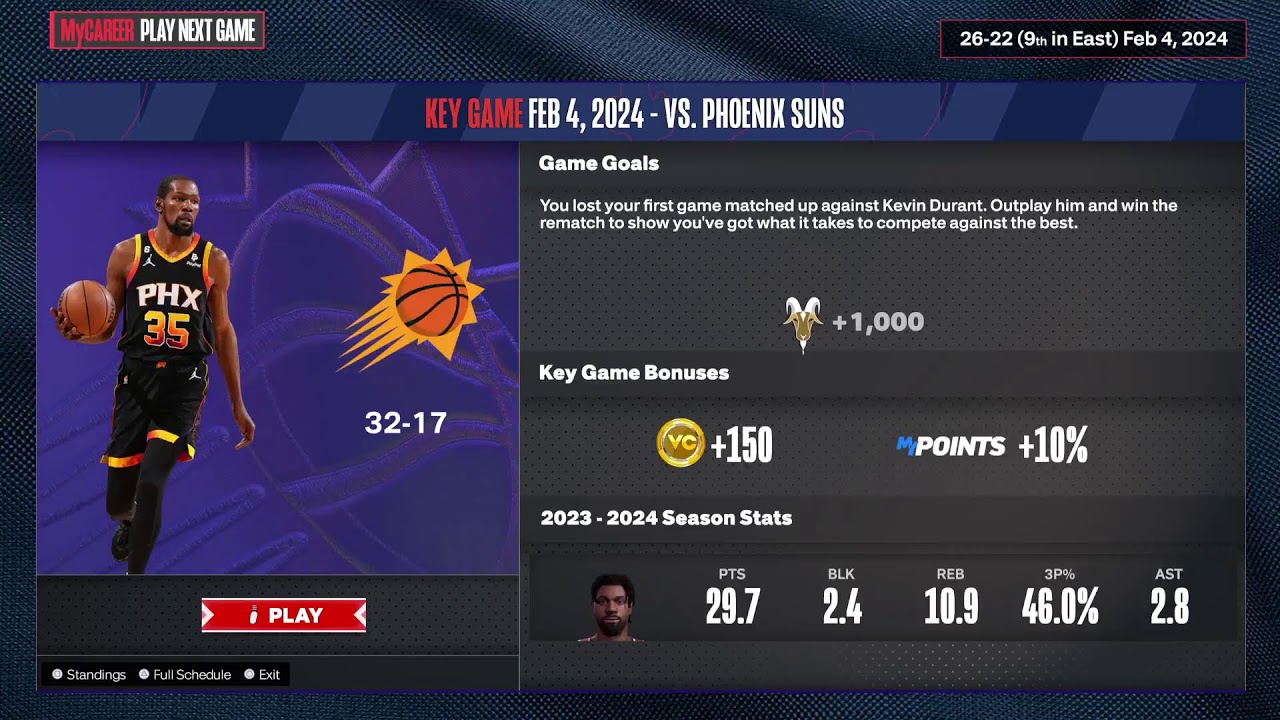The screenshot appears to be from a video game, designed with a sleek black and gray background. In the upper left corner, there is a box displaying red text that reads, "My Career," accompanied by white text to its right that says, "Play Next Game." In the upper right corner, a black box features white text indicating the standings and date: "26-22, 9th in East, February 4th, 2024."

Centered below, there is a highlighted section labeled "Key Game" with the same date, "February 4th, 2024," and shows the upcoming matchup against the Phoenix Suns. On the left side of the screen, an AI-generated image of an African-American basketball player is prominently displayed. The player is holding a basketball and is dressed in a black uniform with distinctive yellow and red ribbing.

The score between two competing teams is shown, reading 32 to 17. Beneath this, a red and white action button is present with the label "Play." At the bottom right of the screen, the text "2023-24 Season Stats" concludes the visual elements of the screenshot.